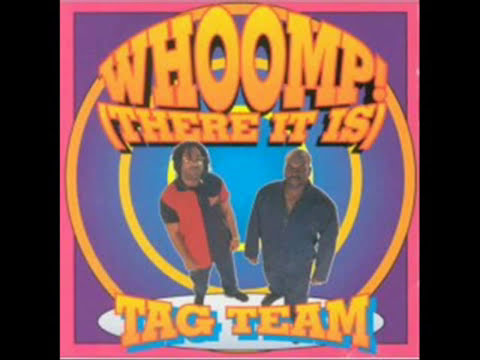The image is a highly detailed album cover for Tag Team's single "W.O.O.M.P. There It Is." The square-shaped cover features a vivid purple background with a pink border. Around the purple background are multiple concentric circles in varying colors: yellow and orange. Positioned centrally within the circles, two men of Tag Team are seen standing and looking up at the camera, shot from a fish-eye perspective. One man wears glasses, has black dreads, and dons a red and black jacket, while the other is bald, without glasses, and wears a black jacket. Both are dressed in black pants. Surrounding them is a blue oval graphic, over which the text "W.O.O.M.P.!" arcs at the top, and beneath the duo is the follow-up text in parentheses, "There it is." At the bottom of the image, under the blue oval, the words "TAG TEAM" are prominently displayed. The left and right sides of the cover are bordered by black rectangles running from top to bottom, further framing the central elements.